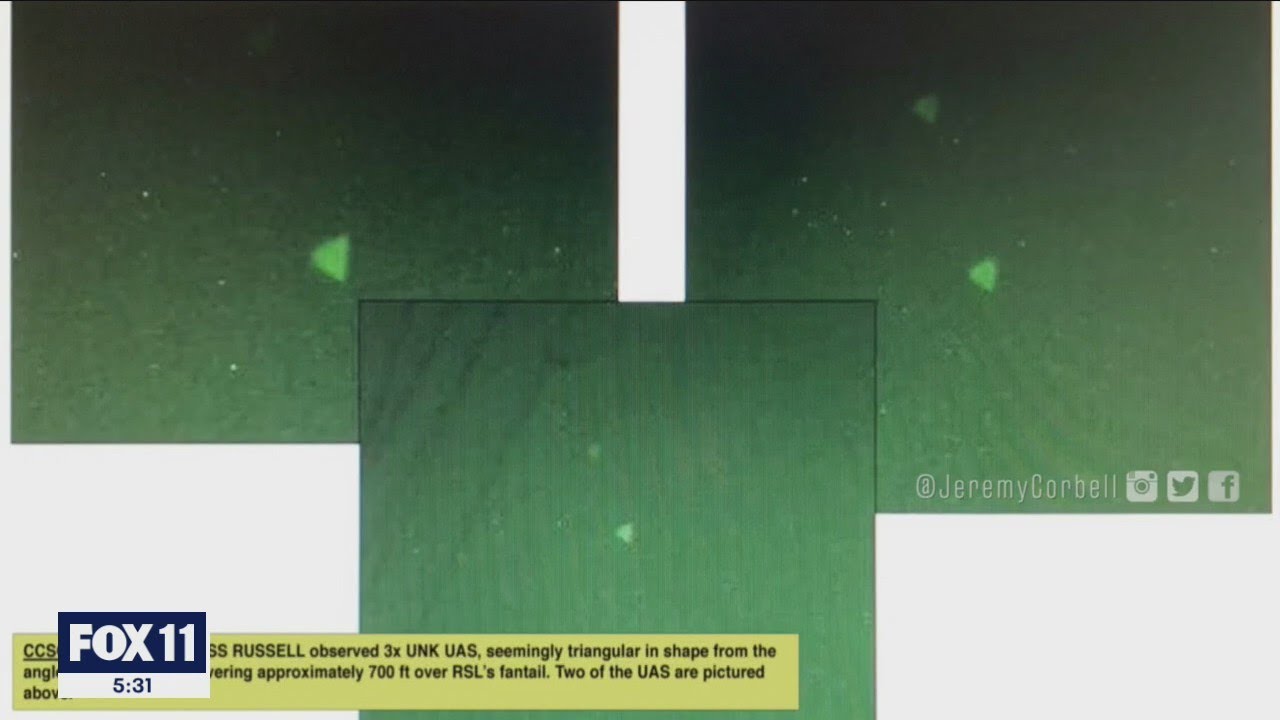The image features three frames set against a very light gray background. The central frame at the bottom displays a gradient green background, transitioning from light green at the bottom to darker green at the top, with a fuzzy white triangular object in the center. Overlapping slightly, the top left frame is larger and depicts a similar scene with a larger image of the white speck. The top right frame, also similar in size to the one on the left, showcases another instance of the white speck, with a gradient from green to black in the top left corner. This top right frame has a watermark on the bottom right that reads "@JeremyKorbel," accompanied by the Instagram, Twitter, and Facebook logos.

The bottom left of the image features a yellow box that partially covers the central green frame. Inside this box is black text, partially obscured, which reads: "Russell observed three times UNK UAS seemingly triangular in shape from the [...] approximately 700 feet over RSL's fantail. Two of the UAS are pictured." Overlapping the yellow box is a white rectangle beneath a blue rectangle. The white rectangle contains smaller blue text "5:31," while the blue rectangle reads "Fox 11" in white text.